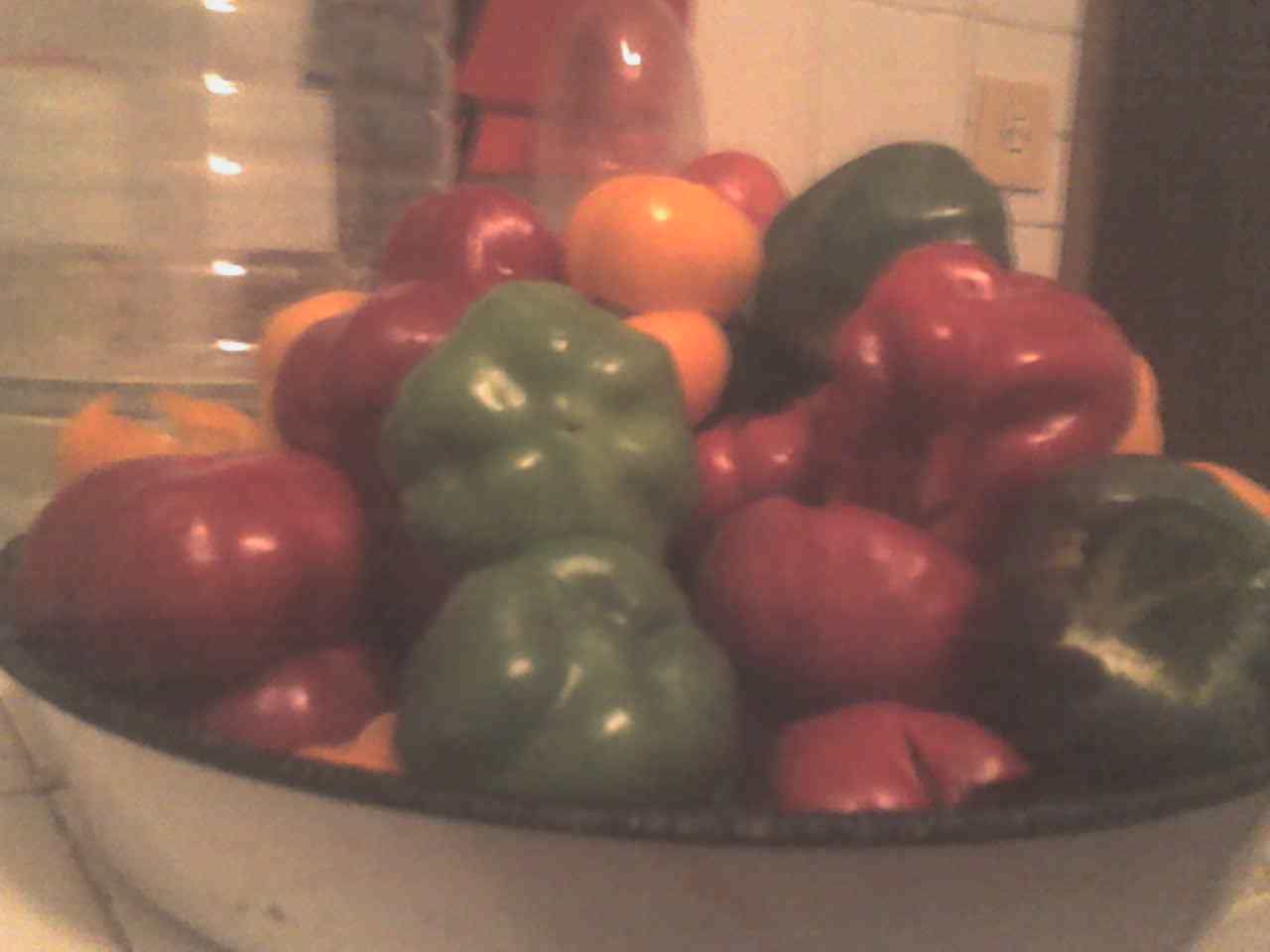This color photograph is a horizontal and rectangular image featuring a slightly blurry and smoky-toned scene. Central to the composition is a creamy white enamel bowl with a black rim, filled to the brim with a variety of vibrant bell peppers – green, red, and yellow. Alongside the bell peppers, there appears to be some red onions or possibly tomatoes. The photograph is dimly lit, likely from a single, dim yellow light source, casting a subdued glow over the scene. In the background, directly behind the bowl, the top of a plastic water bottle is visible, alongside another indistinct plastic object to its left. Further back, a cream-colored light switch is mounted on a wall adorned with white tiles, and what seems to be a black door or doorway is also faintly visible. The overall scene is somewhat obscured, as if taken in motion or through a hazy lens, adding to the atmospheric nature of the photograph.